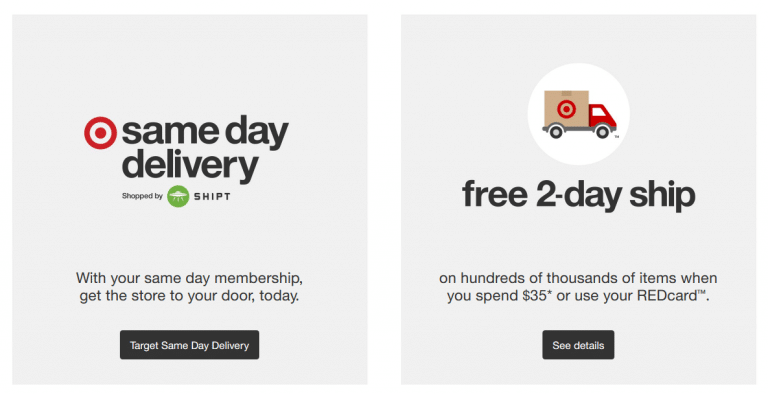This image showcases two promotional screens from Target, both with a light gray background. 

On the left screen, the prominent Target logo, featuring a red circle with a red dot at the center (a red bullseye), stands out. It advertises "Same Day Delivery" in bold white letters, followed by the statement "Shopped by Shipt," accompanied by a green UFO logo. The text further informs customers that with their same day membership, they can get their order delivered to their door on the same day.

The right screen displays an illustration of a delivery box truck bearing the Target logo, encased within a white circle. It promotes "Free 2-Day Shipping on hundreds of thousands of items when you spend $35 or use your RedCard." Beneath this text, there is a "See Details" button for customers to click for more information.